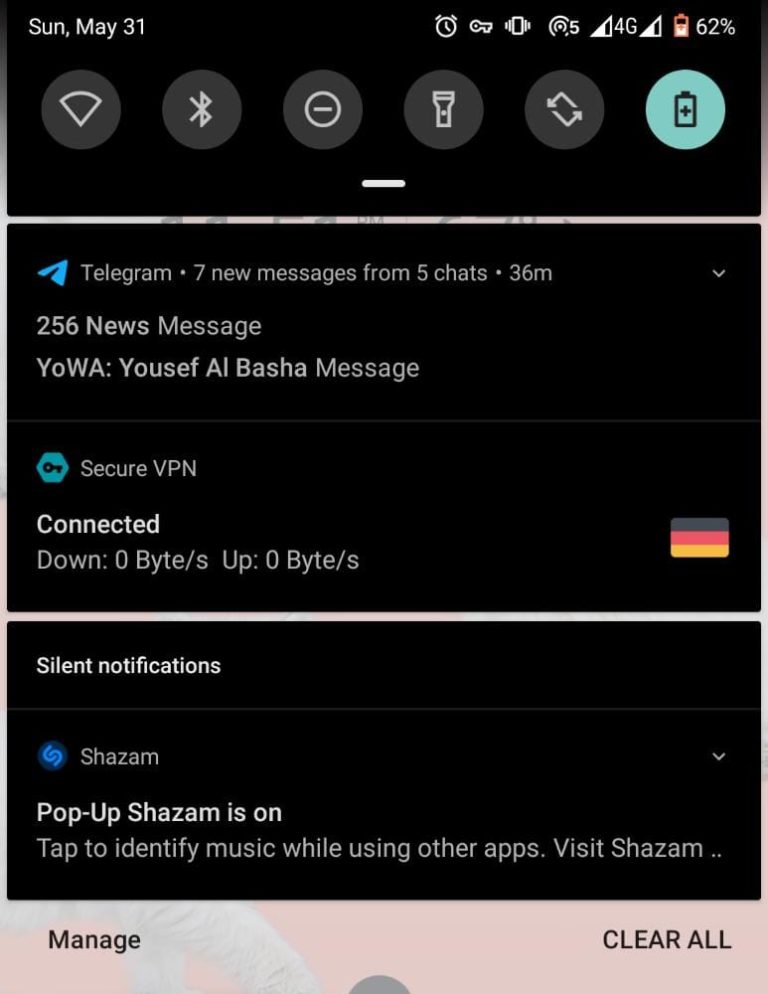Screenshot from a cell phone displaying various status indicators and notifications. At the top left, the date is shown as Sunday, May 31st. On the top right, there is a series of icons: an alarm clock, a key, a vibration symbol, a 4G network indicator, and a battery icon showing 2% remaining. Below this row, additional icons for the Internet, Bluetooth, flashlight, and battery are visible.

In the notifications section, the Telegram app shows 7 new messages from 5 different chats received 36 minutes ago, along with a tally of 256 unread messages. Notifications also include a message labeled "Yawa, Yourself, Albasha," along with a status update from a secure VPN indicating that it is connected, with no data uploaded or downloaded. Silent notifications from Shazam indicate the app is active and ready to identify music, prompting the user to tap for music identification while using other applications.

At the bottom of the screen, in a light pinkish color, two buttons are displayed: "Manage" on the left and "Clear All" on the right. The overall background of the screenshot is black with white text and white lines separating the different sections.